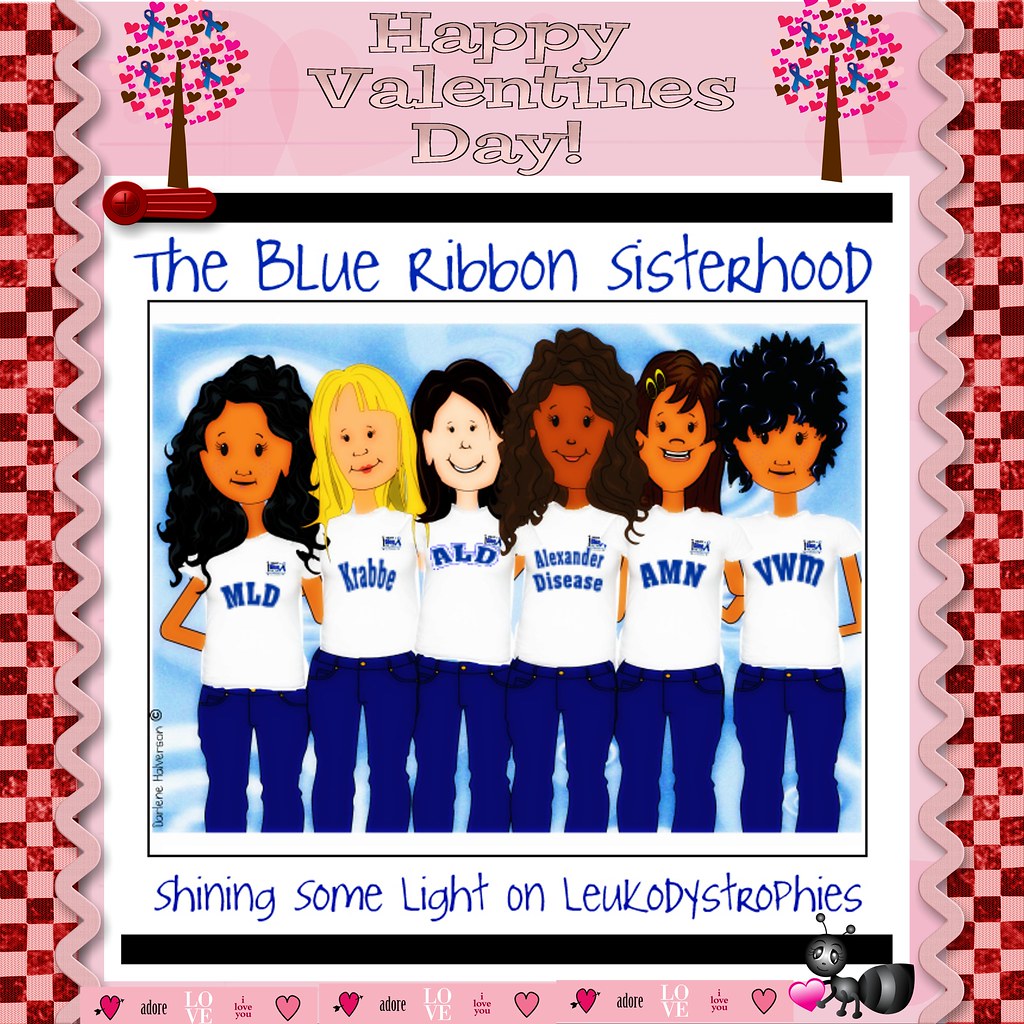This digital art piece celebrates Valentine's Day with an intricate and heartfelt design. At the top, "Happy Valentine's Day" is elegantly inscribed in pink gradient letters that transition to a lighter shade as they descend. Flanking this joyful message are two whimsical trees adorned with heart-shaped leaves and delicate blue ribbons, standing against a rich pink, checkered background accentuated by a zigzag pink border.

Below, a supportive message reads "The Blue Ribbon Sisterhood," followed by "Shining some light on Leukodystrophies," encapsulating the piece's theme of awareness and solidarity. Central to the illustration is a charming depiction of six diverse women, each wearing a white T-shirt personalized with names or initials relating to various medical conditions: "LMD," "Krabbe" (K-R-A-B-B-E), "ALD," "Alexander Disease," "AMN," and "BWM." These women, representing different ethnicities—ranging from brown-skinned to whitish-skinned and Asian—stand united in a powerful illustration of support and community.

At the bottom of this vibrant banner, there's an endearing ant holding a heart, surrounded by additional hearts bearing affectionate messages like "Love," "Adore," and "I love you," adding to the artwork's warmth and charm.